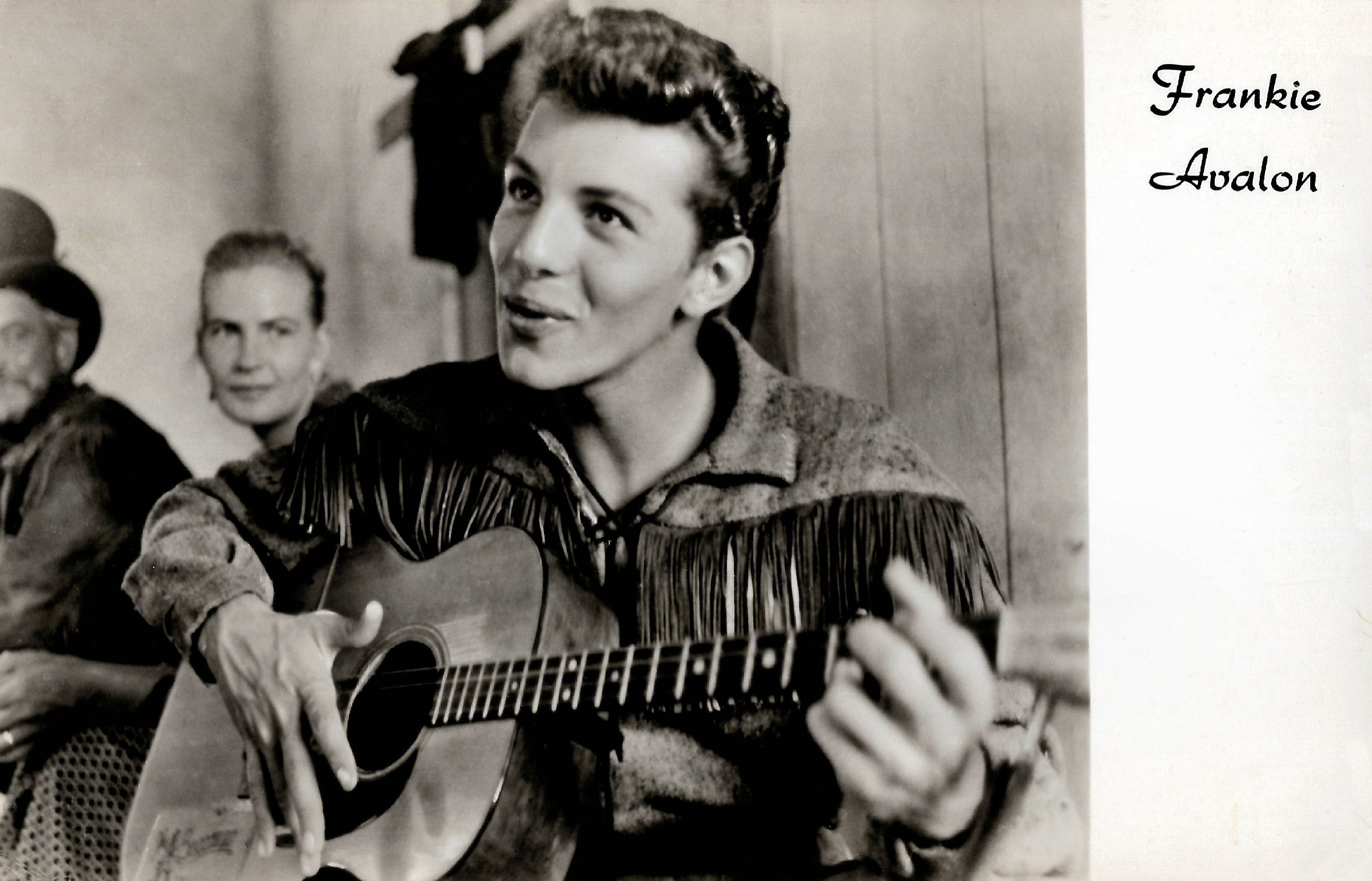In this detailed black and white photo, three individuals are seated on a bench in front of a paneled wall with a central window. The focal point of the image is the person in the middle, whose gender is ambiguous. This individual has short hair styled with volume on top or, if female, hair that might be pulled into a bun. They are dressed in a distinctive buckskin shirt adorned with fringe and are engrossed in singing and playing a small guitar, which has an unfocused sticker on it.

To their left sits a woman with her hair pulled back, dressed in an attire that either consists of a dress or a matching skirt and top featuring a light background with small black diamond patterns. Her hands rest neatly in her lap, and her gaze is directed toward the person with the guitar. On the far left of the bench is a man sporting a black top hat and a mustache, adding to the vintage feel of the photo. Notably, the top right corner of the image is inscribed with the name "Frankie Avalon," anchoring the scene in a specific cultural or historical context.